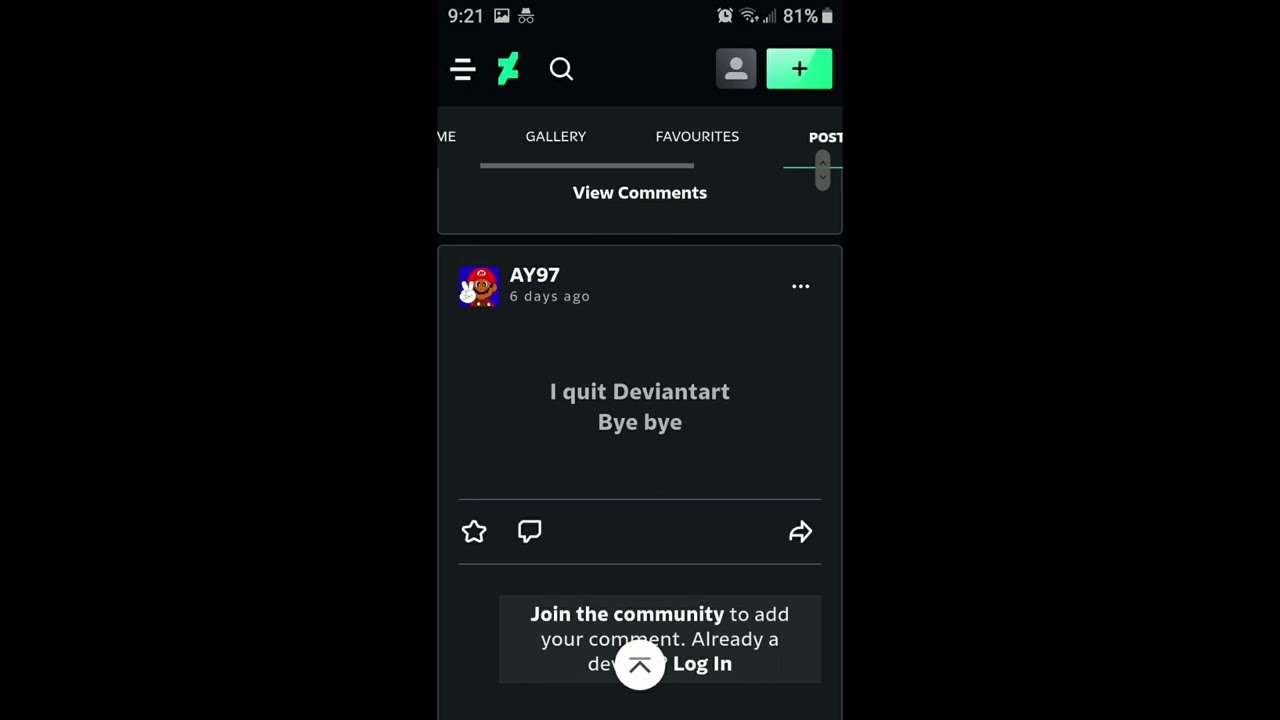This screenshot captures an overlapped interface of a computer screen and a cell phone display. In the top left corner, the time is shown as 9:21, along with a series of small, unidentified icons. On the right side, familiar icons are visible: an alarm clock, a Wi-Fi signal, a weak cell phone signal, a battery displaying 81% charge, and a battery icon.

On the next row, a traditional hamburger menu consisting of three horizontal lines is displayed next to an unspecified logo and a search icon. Beside these, there's a people icon and a clickable green box with a plus sign. Partially visible beneath this row, one can see the letters "M-E," likely part of the word "HOME," followed by the navigation labels "Gallery Favorites," "Posts," and a command to "View comments" delineated by a line.

Directly below is a thumbnail image featuring Super Mario. To the right of this image, the username "AY97" is shown alongside the timestamp "six days ago" and a menu indicated by three horizontal dots. The post content reads, "I quit deviant art, bye bye." Below the post text, there are interaction options with buttons for starring (like), commenting, and forwarding (sharing), represented by a star, a speech bubble, and an arrow icon, respectively. 

At the bottom of the screenshot, a prompt encourages user engagement with the message, "Join the community to add your comment." An additional note for existing members reads, "Already a..." followed by an obstructed word, possibly "login," partially hidden by a circular icon with an upward-pointing arrow.